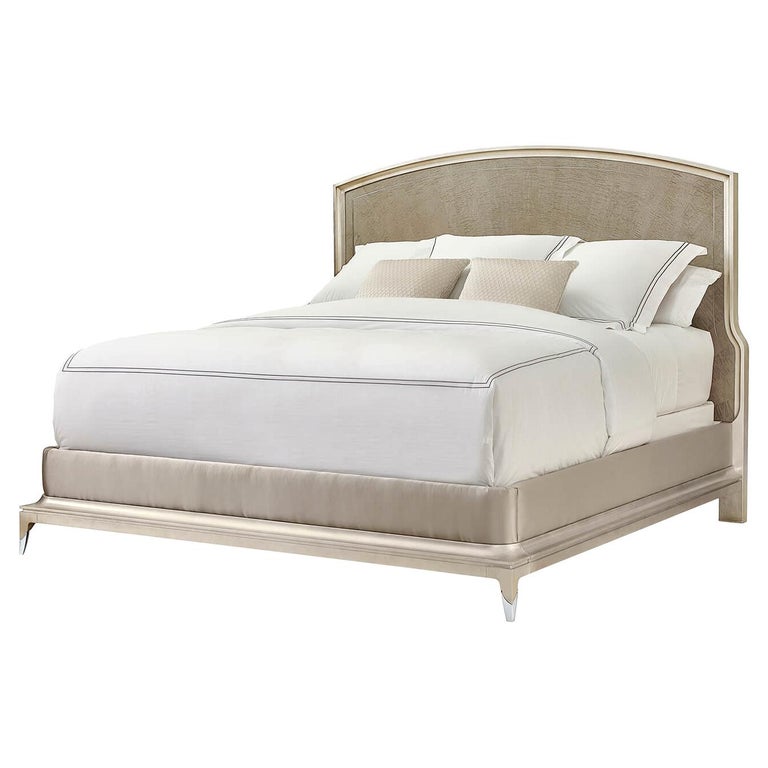This image showcases a meticulously made bed, resembling a double or potentially a king-size, rooted in modern design. The bed features a predominately white comforter with black lining around the edges, accompanied by a set of white pillows with similar black accents. Adding a touch of contrast, there are two decorative light brown pillows in the center. The headboard stands out in a brown wood tone with a lighter beige fabric trim, which gently rounds at the center for a sleek, upholstered look. The bed, probably being showcased for sale online or in a furniture store, sits on four legs: the front legs are beige with silver tips, while the rear ones are sturdier and of a wood beige color. The entire bedding ensemble is expertly tucked in, exposing the feet of the bed and maintaining a pristine appearance. The simplicity in its background highlights the bed's comfort and style, with an overall color palette of white, beige, and brown, conveying a serene and inviting atmosphere.